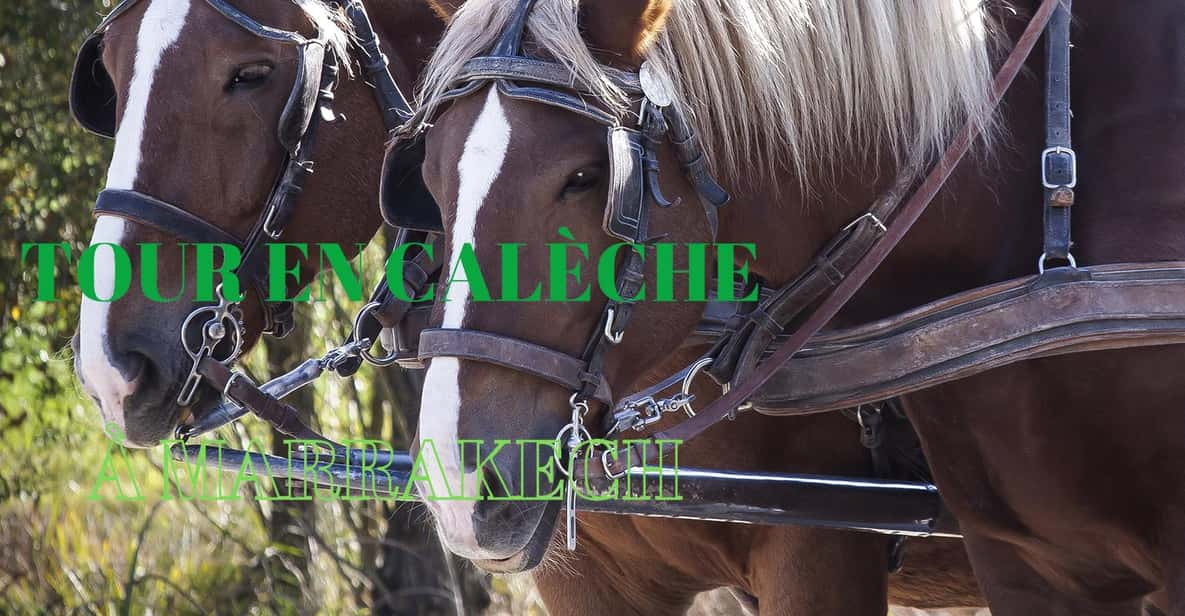In this close-up image, two chocolate brown horses are shown outside, captured from the shoulders up. Both horses are equipped with similar bridles featuring a leather strap around their noses and another around their heads, suggesting they are part of a team, possibly harnessed to a carriage or plow. The horse closest to the viewer stands out with a distinct white mane and a white streak running from its forehead to its nose. The second horse, positioned to the left, also has a white stripe on its forehead, although the end of its nose is not visible. The background reveals some long, wild grass in the bottom left corner. Overlaying the picture, there's text in a green font that reads "U-R-E-N-C-A-L-E-C-H-E" with an additional, partially obscured word beneath it.